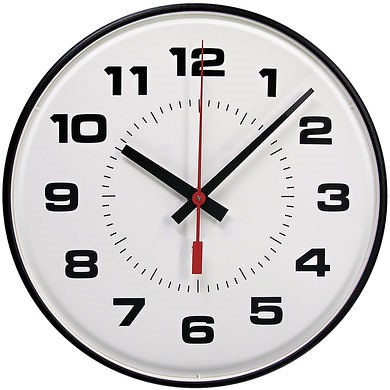This detailed close-up image features a classic, circular wall clock commonly found in schools. The clock has a plain black frame and a white face, with black numerals from 12 to 11 arranged in a standard clockwise formation. The hour and minute hands are black, while the second hand is red. At the time captured in the image, the hour hand is slightly past the 10, the minute hand is between the 1 and 2, indicating approximately 10:08, and the red second hand is slightly past the 12. The clock also features a smaller circle inside the main face delineated with black hash marks representing every minute, and thicker marks at every hour position. The background of the image is white, further emphasizing the contrast and clarity of the clock's features. The hands are held together by a small silver pin at the center.